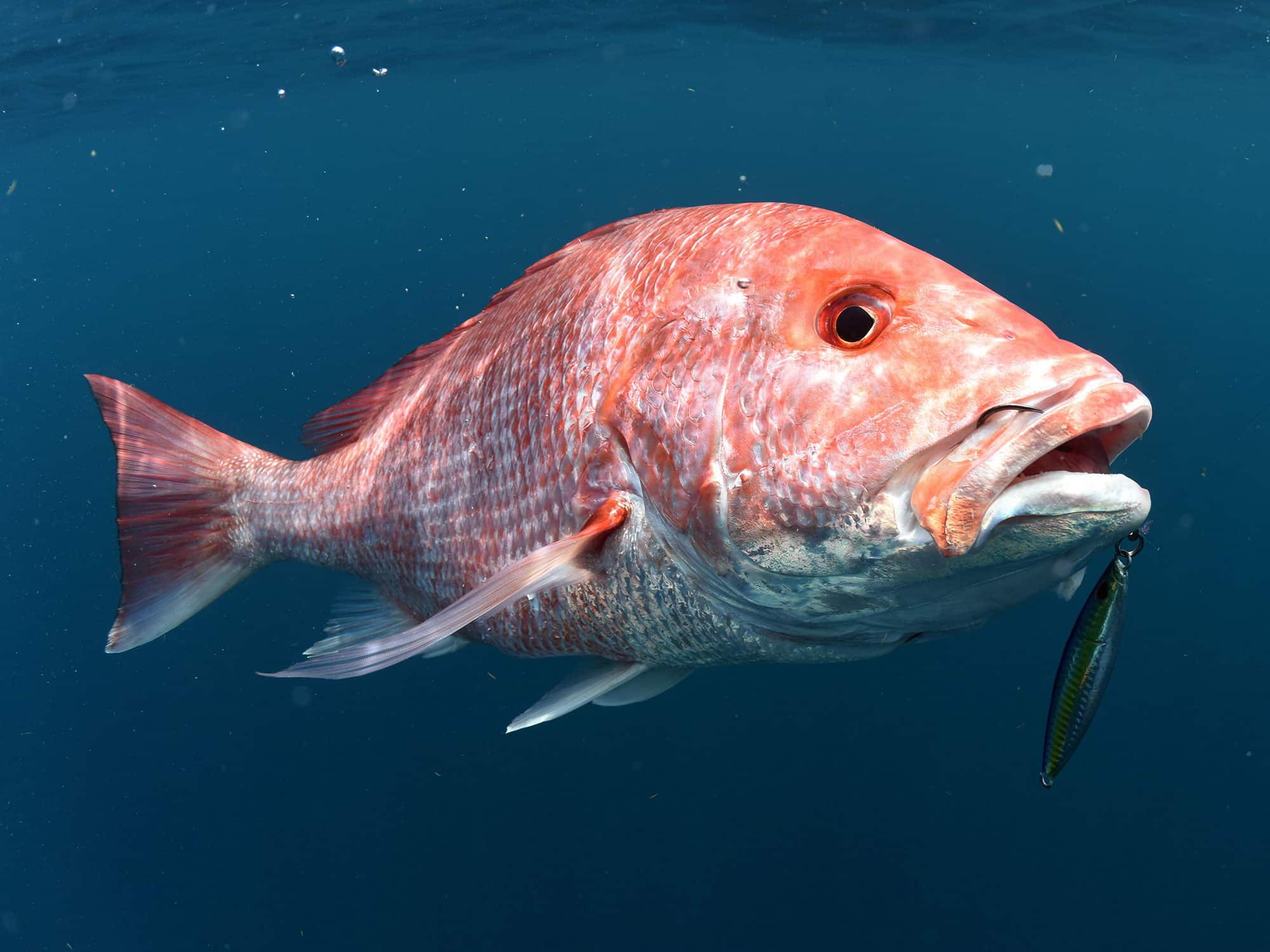The image captures a close-up scene of a fish underwater. The fish is primarily light orange with a gradient to white on its underside, particularly its belly. Positioned with its right side facing the camera, the fish reveals only its right eye, which appears as a black dot. The background features water in varying shades of blue, darker at the bottom and lighter towards the top. The fish is adorned with fins on both its top and sides, which are a mix of pinkish and white hues, with the bottom fins displaying a whitish, translucent quality. A metal fishing lure is hooked into its mouth, emerging from the upper lip on the right side and hanging from the bottom lip on the left. This lure is oval-shaped, primarily dark green with a silver top and bottom, mimicking a small fish. The image emphasizes the unfortunate situation of the fish possessing this lure in its mouth, indicating it might have had an encounter with a fisherman. Overall, the fish's coloration, and detailed lure create a vivid underwater scene against the dark blue aquatic background.